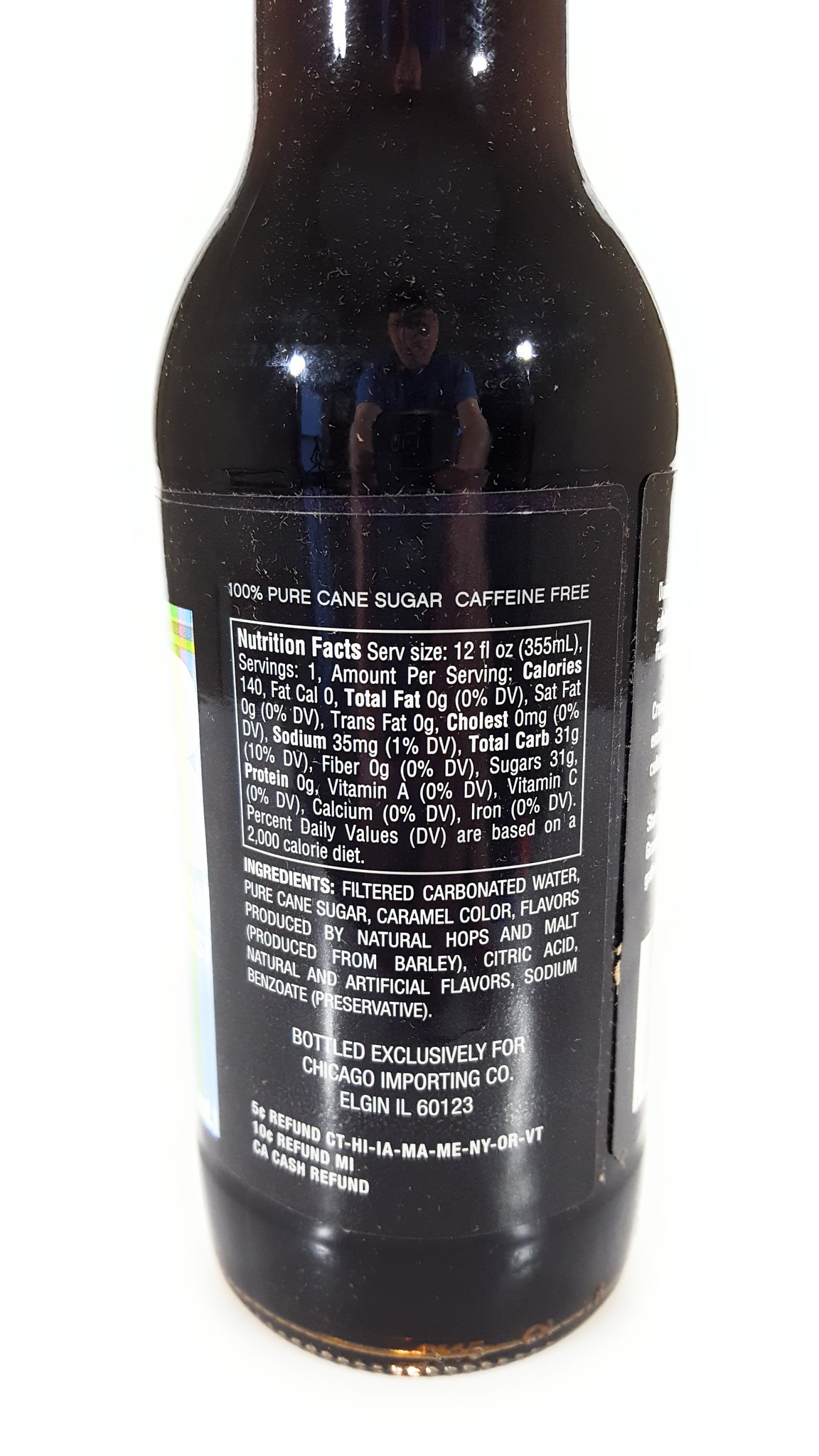This detailed photograph features a close-up view of a dark-colored cola bottle, slightly dusty or pitted, and vertically oriented. Prominently displayed in white text on the brown label at the top, it reads "100% pure cane sugar, caffeine-free." The bottle's label details both the nutrition and ingredients information. The nutitional facts, presented in a rectangular box with a white border, indicate a serving size of 12 fluid ounces (one serving) containing 140 calories, 0 calories from fat, 0g total fat, 0g saturated fat, 0g trans fat, 35mg sodium, 31g total carbohydrates, 0g dietary fiber, 31g sugars, and 0g protein. Additionally, the ingredients are listed as follows: filtered carbonated water, pure cane sugar, caramel color, flavors produced by natural hops and malt from barley, citric acid, natural and artificial flavors, and sodium benzoate (preservative). The bottle was bottled exclusively for Chicago Importing Company, located in Elgin, Illinois, 60123. Notably, there is a reflection on the bottle showing a person wearing a short-sleeved blue shirt, with visible forearms being the only distinguishable features.